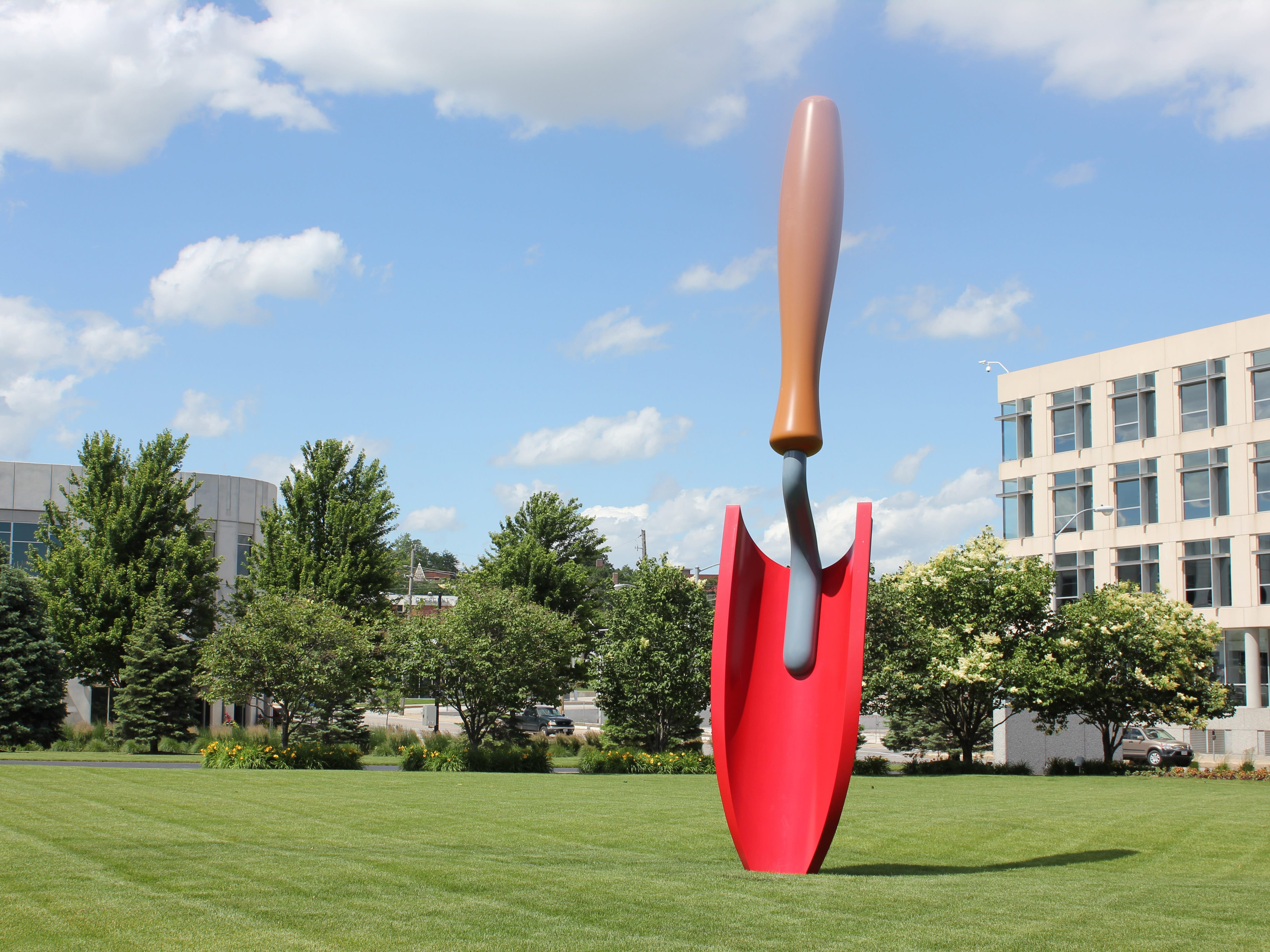This photograph showcases a striking outdoor art installation set in a park within a business district. The central feature is an enormous sculpture of a gardening trowel. The trowel has a red blade, a gray shaft, and a brown handle, and it is plunged into the green lawn as if someone had just paused while gardening. The surrounding park area is flanked by several office buildings, including a prominent white building with multiple floors and numerous windows. Cars can be seen parked along the adjacent road. In the background, there are trees lining the park, which are not as tall as the four-story office buildings, standing at an estimated 25 to 30 feet. The image captures a bright, sunny day with a clear blue sky adorned with puffy white clouds. The sunlight bathes the entire scene, enhancing the vibrant colors and the detailed textures of the sculpture and its surroundings.